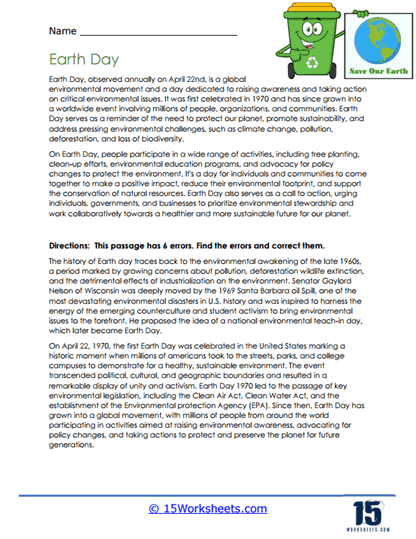This detailed description serves as a cleaned-up and elaborated caption for the image:

---

**Earth Day Educational Worksheet from 15worksheets.com:**

At the top of this Earth Day-themed worksheet, designed for educational use, there is a space for students to write their names, located in the upper left corner. On the upper right corner, a cheerful green recycling bin with arms is illustrated, pointing to a vibrant drawing of the Earth, colored in shades of blue and green. The recycling bin's lid is highlighted in yellow, and it prominently displays the message "Save Our Earth."

Just beneath this illustration, the worksheet’s title "Earth Day" introduces two detailed paragraphs. The first paragraph provides the history of Earth Day, enriching students with background information about the environmental movement. The second paragraph explores various ways people participate in Earth Day activities, emphasizing community involvement and sustainability practices.

Following the informational content, a bolded directive states: "Directions: This passage has six errors. Find the errors and correct them." Below this instruction, the original content of the two paragraphs is repeated but rewritten with intentional errors for students to identify and correct as a grammatical and comprehension exercise.

A blue line runs horizontally across the bottom of the page, marking the end of the content and providing a neat conclusion to the worksheet.